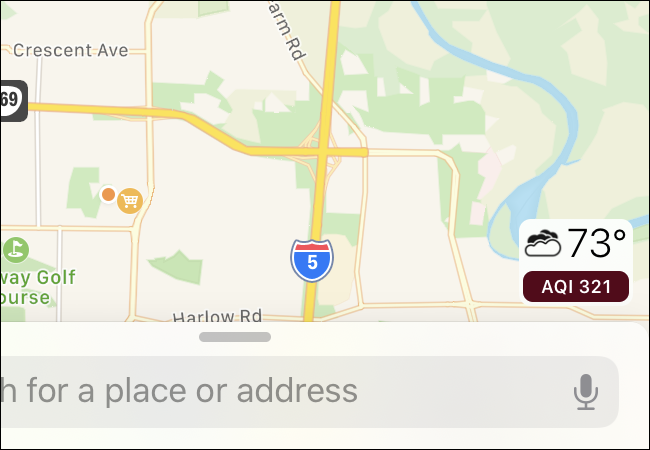This detailed caption is for an image of a Google Maps interface displayed on a mobile phone screen:

The image shows a Google Maps interface on a mobile phone. At the bottom of the screen, there is a search bar with the text, "Search for a place or address," accompanied by a small microphone icon for voice search. The current temperature is displayed as 73 degrees, and the Air Quality Index (AQI) is marked at 321. The map prominently features major routes such as Route 5 and Route 69. Noteworthy locations on the map include a golf course, Harlow Road, and Crescent Avenue. A river is also visible, represented by a blue water feature. In addition, a shopping center is indicated by a yellow shopping cart icon. There are patches of light green on the map, denoting green spaces. Furthermore, 'Arm Road' is listed as one of the streets. Major routes are highlighted in bright yellow. The weather appears to be partly cloudy with the temperature at 73 degrees.